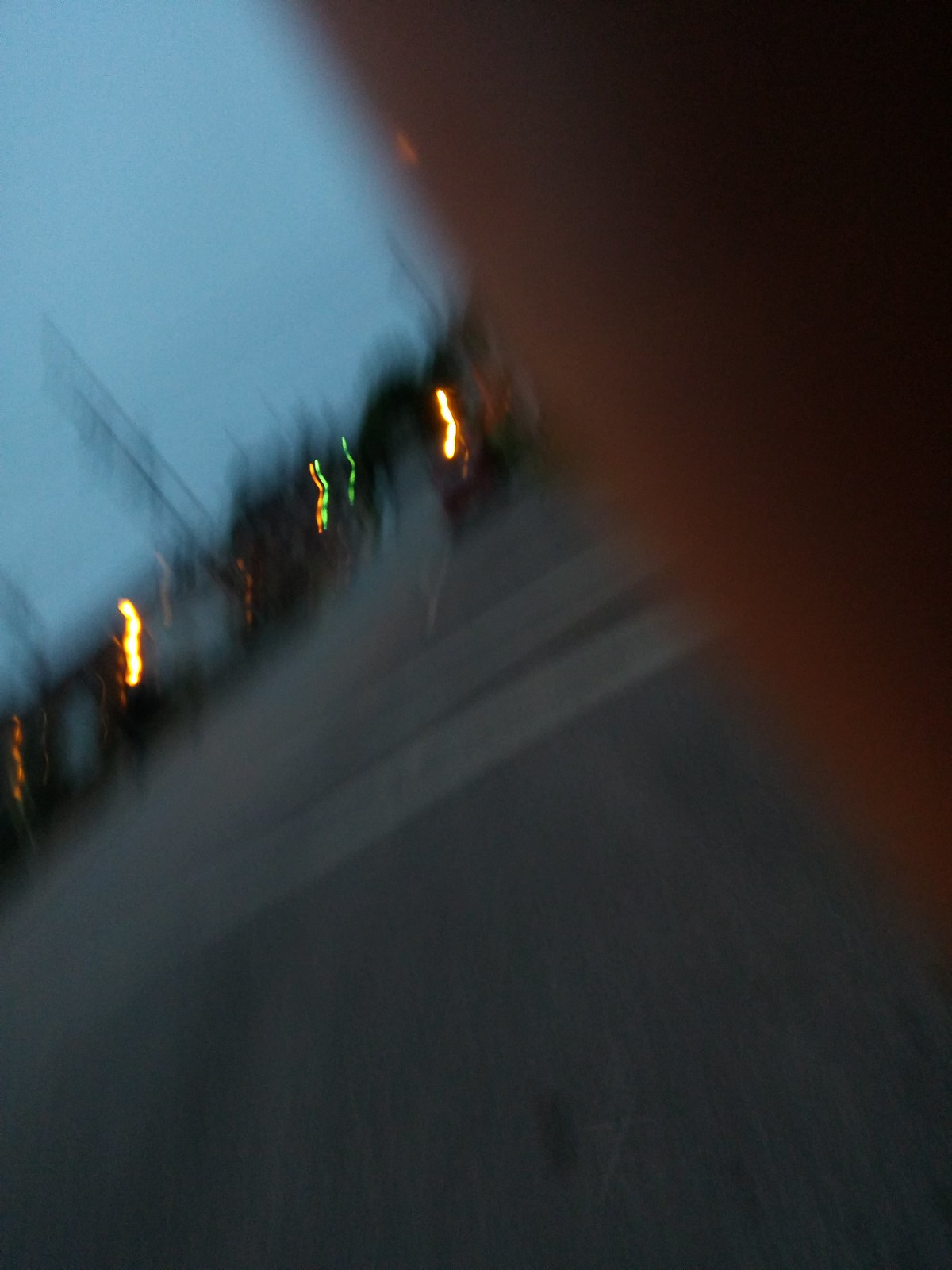This is an extremely blurry photograph, likely taken with a phone in portrait mode while the person was moving, possibly biking or walking, which contributed to the heavy blurriness. The image is partially obscured by a finger covering almost half of the lens on the right side. The visible portion of the image reveals a street scene at dusk, with the sun already set, casting a darker ambiance. There are several orange and green lights that appear dragged across the screen due to the motion, and these lights suggest nearby cars and street lamps. The upper left-hand corner shows a faint, sideways view of a light blue sky. The street includes a crosswalk and some macadam, with vague outlines of utility poles and indistinct structures or buildings in the background. There appears to be one car in the right lane ahead, near the middle of an intersection, and the entire scene hints at an outdoor environment, likely a parking lot or street area.